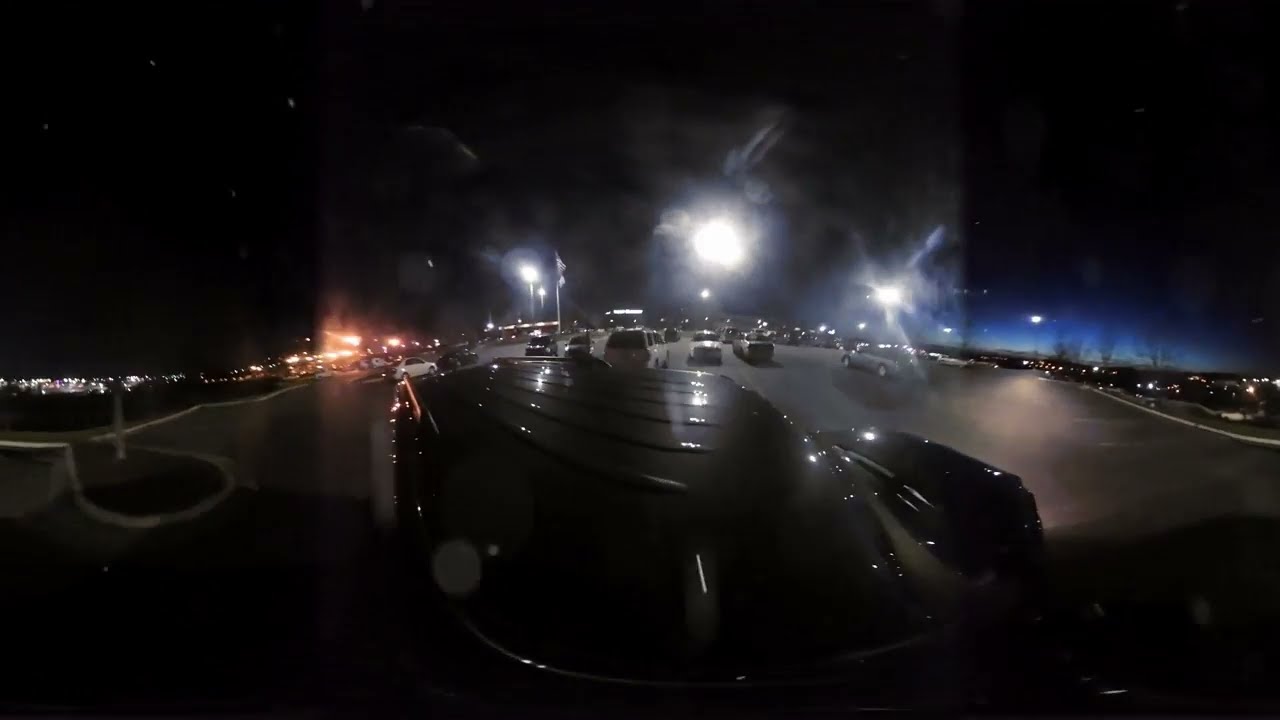The image captures a dark, nighttime scene of a parking lot with a horizontal rectangular shape. The top portion of the image is dominated by an inky black sky, providing a stark contrast to the dimly lit parking lot below. The center of the image features several parked cars, including white SUVs and gray trucks, resting on a gray cement surface. Amidst the vehicles, a prominent black car with a flat roof and a futuristic design stands out, somewhat resembling a Batmobile. Sparse lighting illuminates parts of the parking lot, casting long shadows and only faintly revealing the surroundings.

On either side of the lot, the scene fades into grayed-out sections that hint at more details. The left side reveals a white curb, green grass, and some bushes and trees, while the right side similarly displays gray streets with white lines, more curbs, and additional lights flickering in the background. Some trees have lost their leaves, appearing as bare brown stems. Far off in the distance, beyond a vast expanse of darkness, city lights twinkle and highlight the horizon, adding depth to the composition and suggesting an isolated, possibly rural setting. There is no text in the image, which immerses the viewer in the silence and stillness of the night.